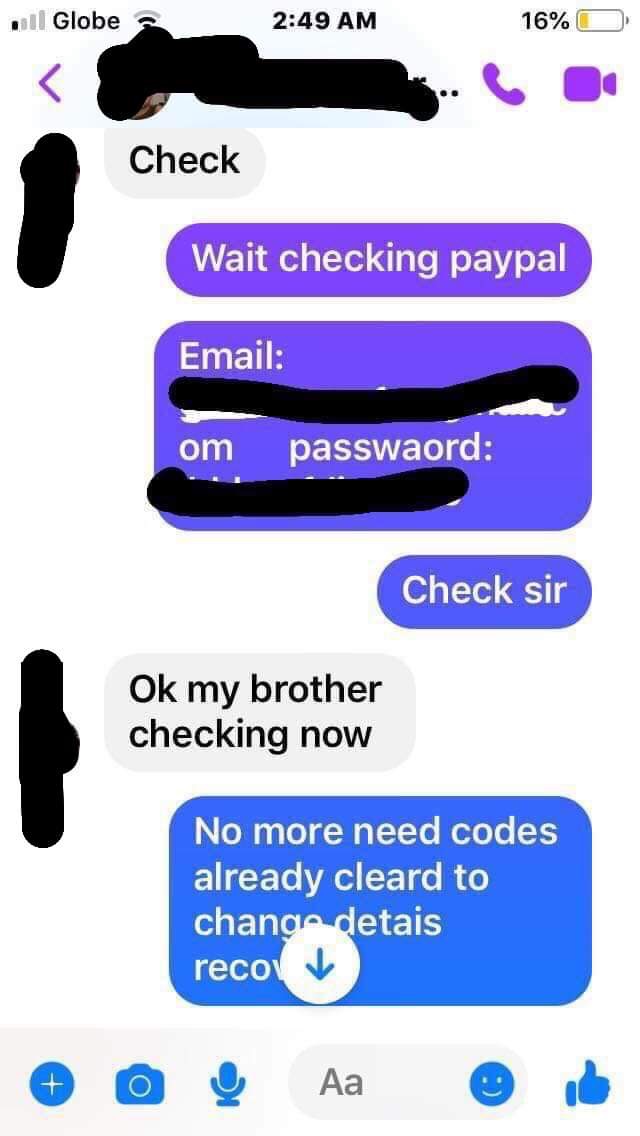This is a detailed screenshot from an iOS device taken at 2:49 a.m., with a battery level of 16%. The top of the screen shows the carrier as Globe, a Philippines-based telecom company. The screenshot displays an ongoing conversation in the Facebook Messenger app, characterized by varying colored bubbles indicating different speakers. The background is white with a purple balloon theme. Some personal information, such as the names and email addresses, are blacked out for privacy.

The sequence of the conversation involves the recipient initially saying, "check," followed by the sender responding with, "wait, checking PayPal." Several sections, specifically the email and password, are crossed out with black lines to maintain confidentiality. The sender continues with, "check sir," to which the recipient replies, "okay my brother, checking now." Finally, the sender assures, "no more need. Code's already cleared to change details. Recovery."

At the bottom of the screenshot, the Facebook Messenger UI is visible, showing options to share media, take a picture, send a voice recording, type a message, or send a thumbs up. This image highlights a meticulous exchange possibly related to verifying or modifying PayPal account details.